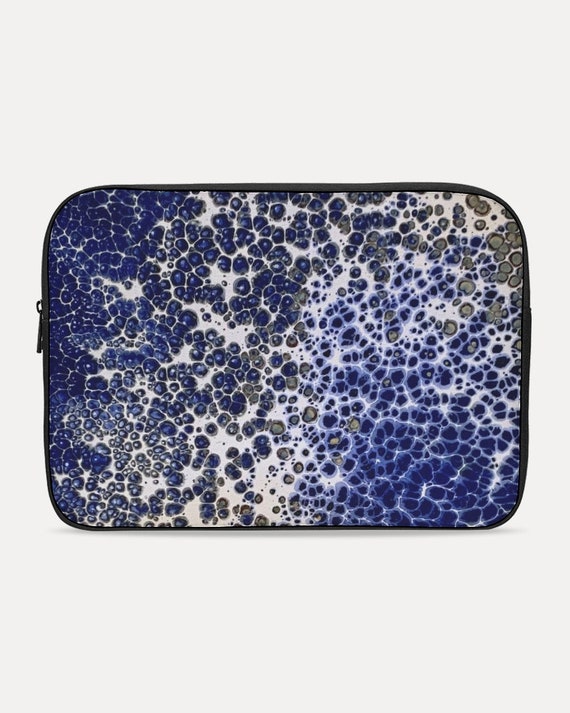The photograph features a side view of a sleek, uniquely-textured purse or wallet set against a solid white background. The accessory is characterized by a shimmering, iridescent surface in shades of metallic blue, accented with speckles and dots in hues of blue, gray, and white. This intricate surface, reminiscent of scales or the texture of a pancake cooked on a griddle, reveals an underlying dark black color through its myriad of tiny pockmarks and holes. Running from the right side of the purse across to the left, a black zipper adds a functional and contrasting detail. The rectangular shape of the accessory, combined with its glossy yet rugged material, intrigues with its visually striking and tactile appeal.